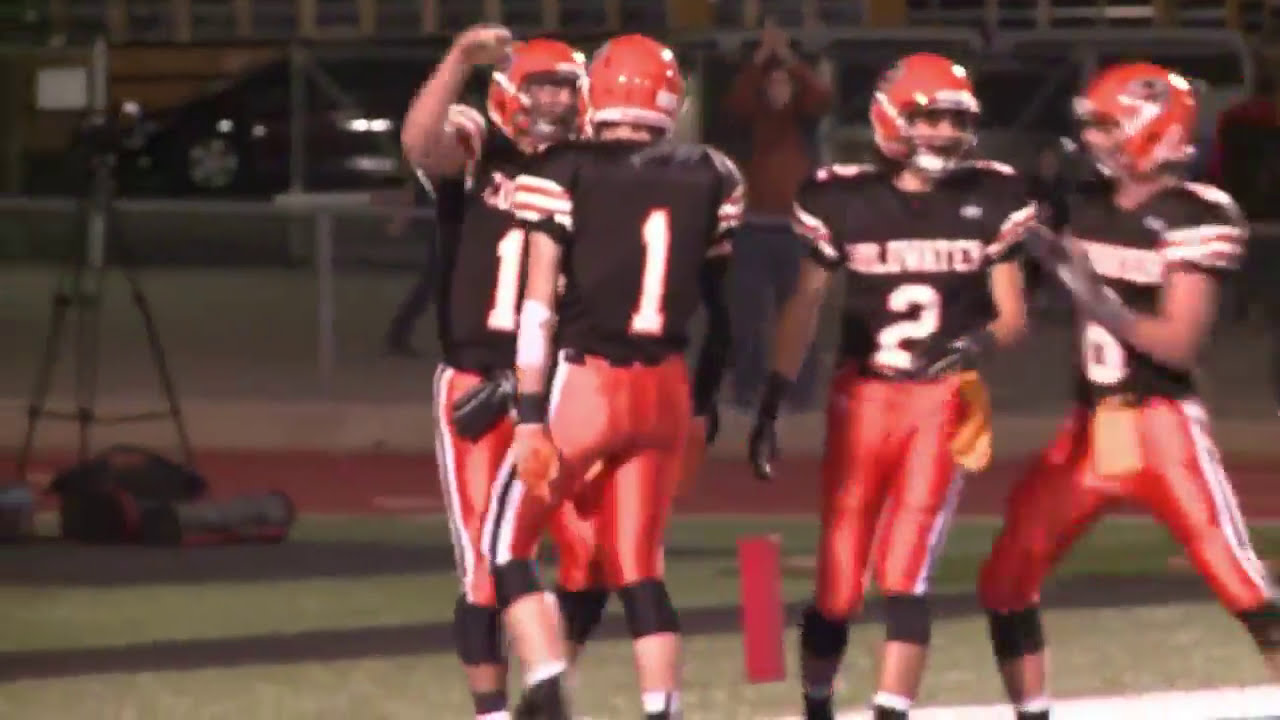In this image, we have a scene from a high school football game, showcasing four football players who appear to be celebrating a touchdown. The players are positioned towards the middle and right-hand side of the wide, rectangular, outdoor image. They are all wearing matching uniforms consisting of black jerseys with white numbers outlined in orange, and red pants with white and black stripes. Their helmets are red, accented with silver. The players are touching and congratulating each other, clearly elated by the recent play. 

The green turf field beneath them shows horizontal gray shadows, indicating bright sunlight. A red track encircles the field, evident better at the bottom and middle parts of the image. Behind the track, a fence demarcates the area, with a parking lot visible beyond it, containing several cars and school buses, further suggesting a high school or middle school setting. On the left side of the track, an object on a tripod stands out. People are present around the field, some clapping and enjoying the game. The overall scene conveys the vibrant energy and communal atmosphere typical of school football games, despite the image being blurry and of low resolution.